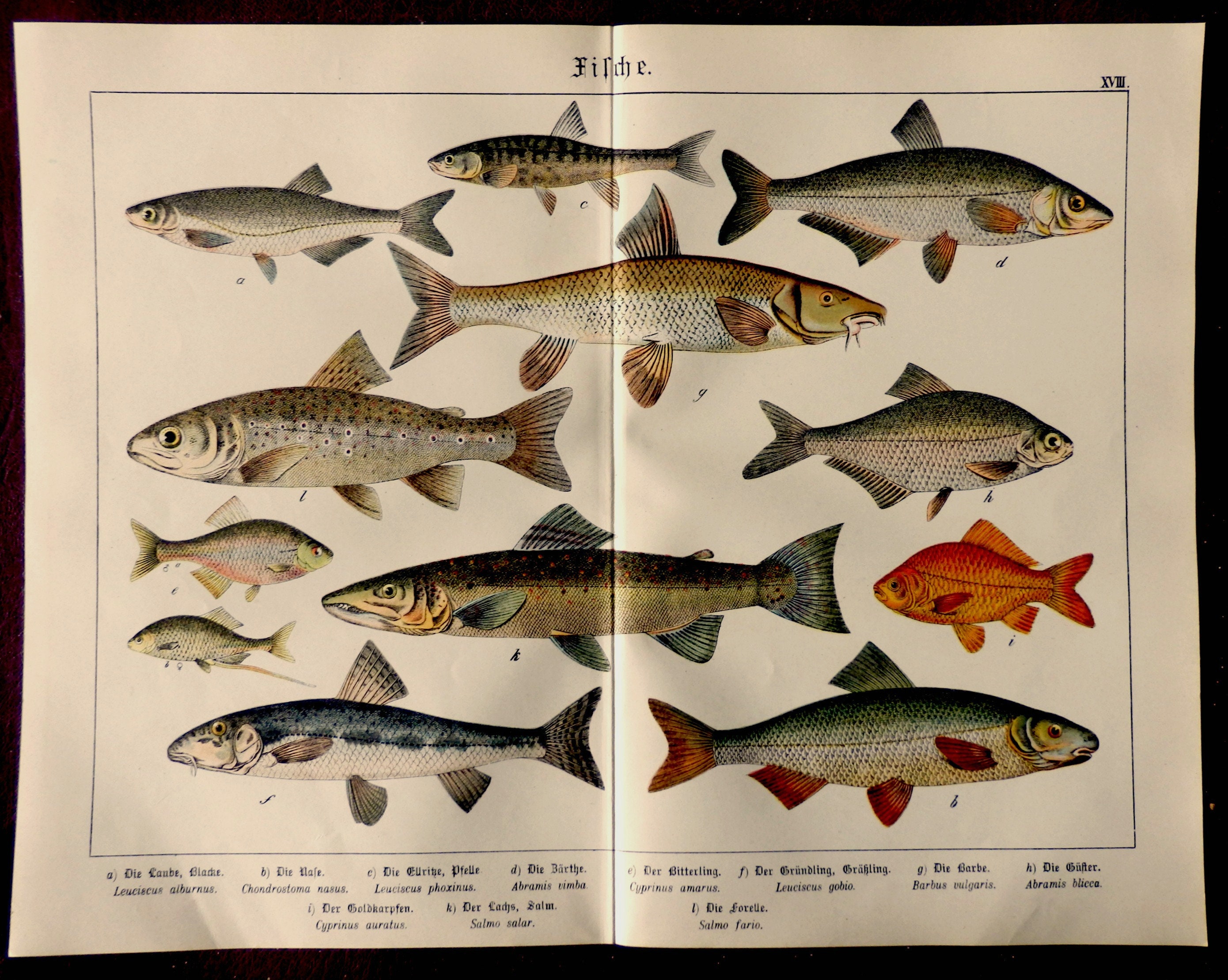This photograph captures an open vintage book displaying a detailed artist's rendition of twelve different species of fish in a double page spread. The fishes are illustrated in side profile, with varying colors, sizes, and distinctive features, meticulously rendered to depict their uniqueness. Most of the fish exhibit grayish-blue hues with subtle hints of yellow, while others boast vibrant shades, including an orange fish on the bottom right, a green and white fish with red gills just above it, and others with red, orange, blue, and pink elements. Their sizes range from small, around three to four inches, to larger specimens exceeding a foot in length. The fish face different directions across the pages, adding dynamic diversity to their presentation. The pages also contain small texts; a key at the very bottom of the spread correlates letters assigned to each fish with their respective species names, though the old English script and diminutive size of the writing make it challenging to read. At the top of the page, there's additional text, possibly in another language, starting with "F-I-L". The scene beautifully blends the artistic illustration with a historic, almost scholarly charm.